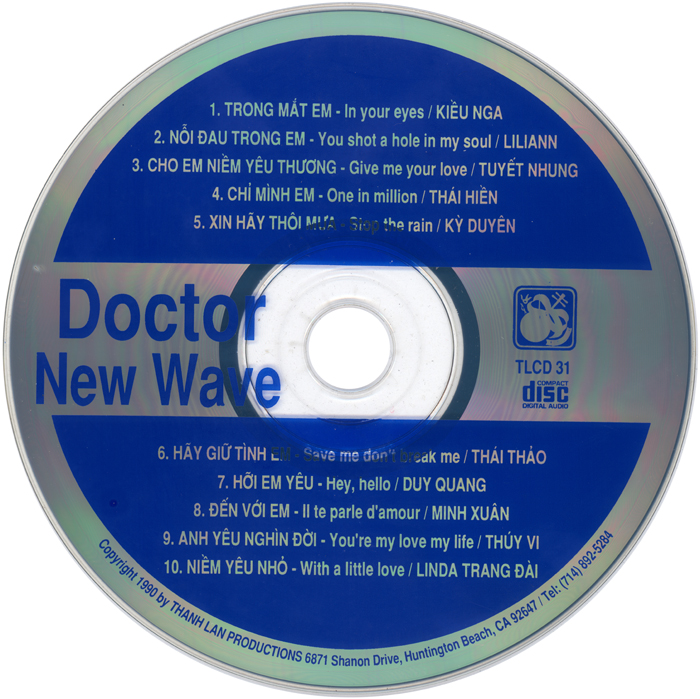This photograph displays a music CD titled "Dr. New Wave," featuring songs listed in both English and another language, which appears to be Vietnamese. The CD, identified as TLCD 31, is produced or copyrighted in Huntington Beach, California. The background of the CD is a blend of blue and gray, with the text printed in white and blue. In the center of the CD, the prominent text "Dr. New Wave" is positioned above the central hole of the CD. Surrounding this title are ten songs, named both in English and Vietnamese. Song number one is "In Your Eyes" (Trong Mat Em), number two is "You Shot a Hole in My Soul," three is "Give Me Your Love," four is "One in a Million," five is "Stop the Rain," six is "Save Me, Don’t Break Me," seven is "Hey Hello," eight is "Parlez de Moi" (in French), nine is "You're My Love, My Life," and ten is "With a Little Love." The photograph distinctly highlights the dual-language track listings and the artistic design of the CD.